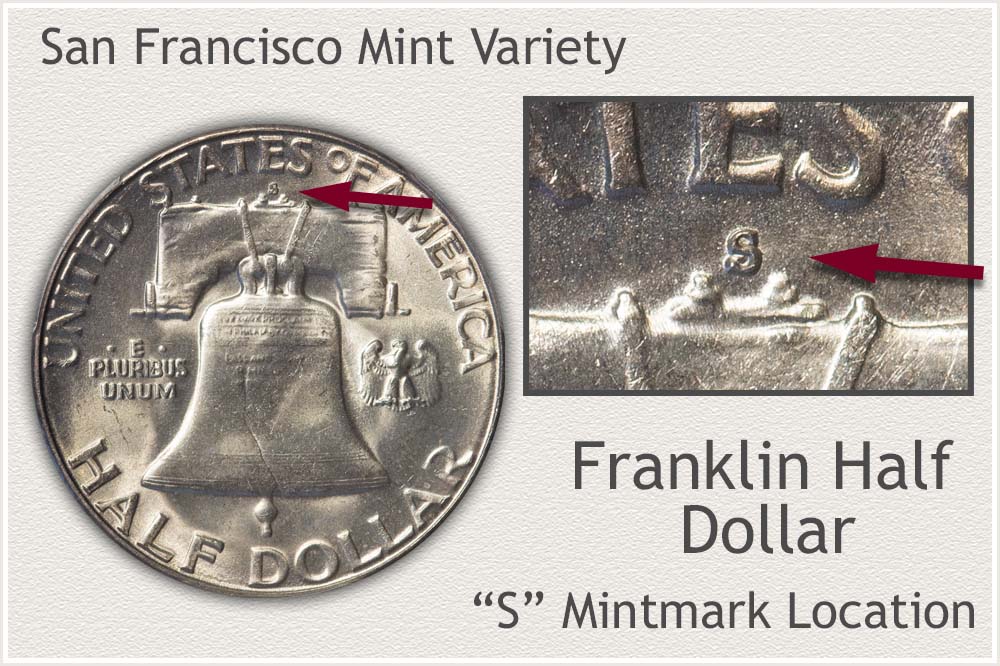The image depicts a highly detailed photograph of a shiny, silver-colored Franklin Half Dollar coin. The coin, placed against a grainy white background, prominently features the inscription "United States of America" and "Half Dollar" around the Liberty Bell. Above the bell, a small "S" mint mark is visible. Overlaying the upper left corner of the image is dark text that reads "San Francisco Mint Variety." To the right, there is a close-up snapshot of the coin's detail with a red arrow pointing to the mint mark above the Liberty Bell. Beneath this close-up, dark gray text states "Franklin Half Dollar 'S' Mint Mark Location."